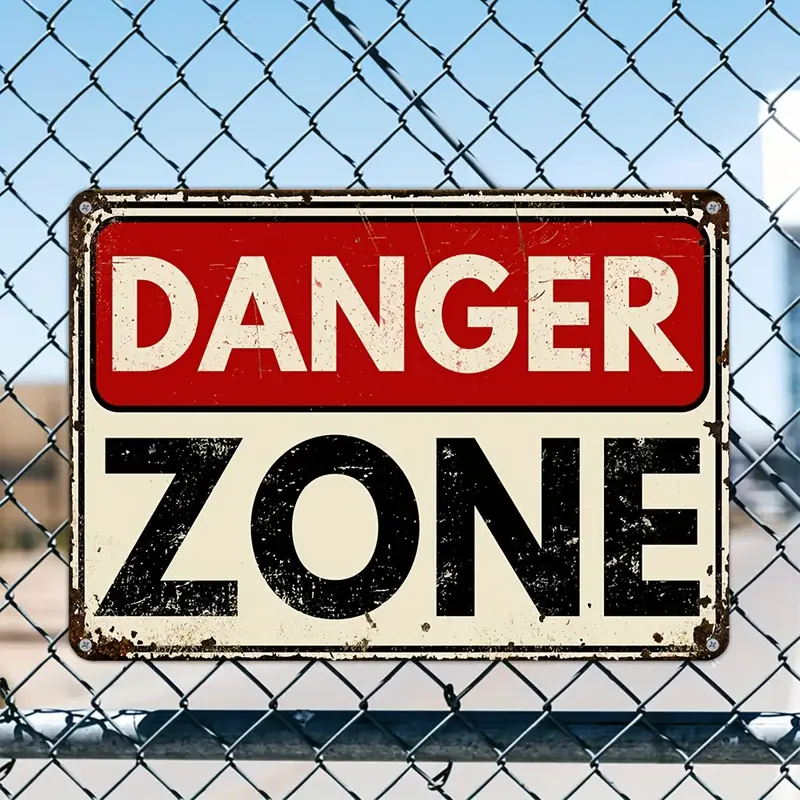This close-up photograph captures a weathered "Danger Zone" sign firmly attached to the middle of a chain link fence with diamond-patterned links. The sign itself features the word "Danger" in white letters on a red rectangular background at the top, while "Zone" is prominently displayed in bold black letters on a white background in the lower half. The sign’s edges show signs of rust and distress, with additional rust spots scattered across its surface, hinting at years of exposure to the elements. Secured with screws at its four corners, the sign has a brown-edged border that further accentuates its aged appearance.

In the backdrop, an unfocused haze of color depicts a bright blue sky, patches of brown land, green foliage, and hints of a parking lot and streetlight, suggesting a vast and open area behind the fence. At the bottom of the image, a silver steel bar runs horizontally, emphasizing the sunny day setting. Overall, the photograph exudes a sense of caution and aged resilience, framed by the sturdy metal links of the fence.